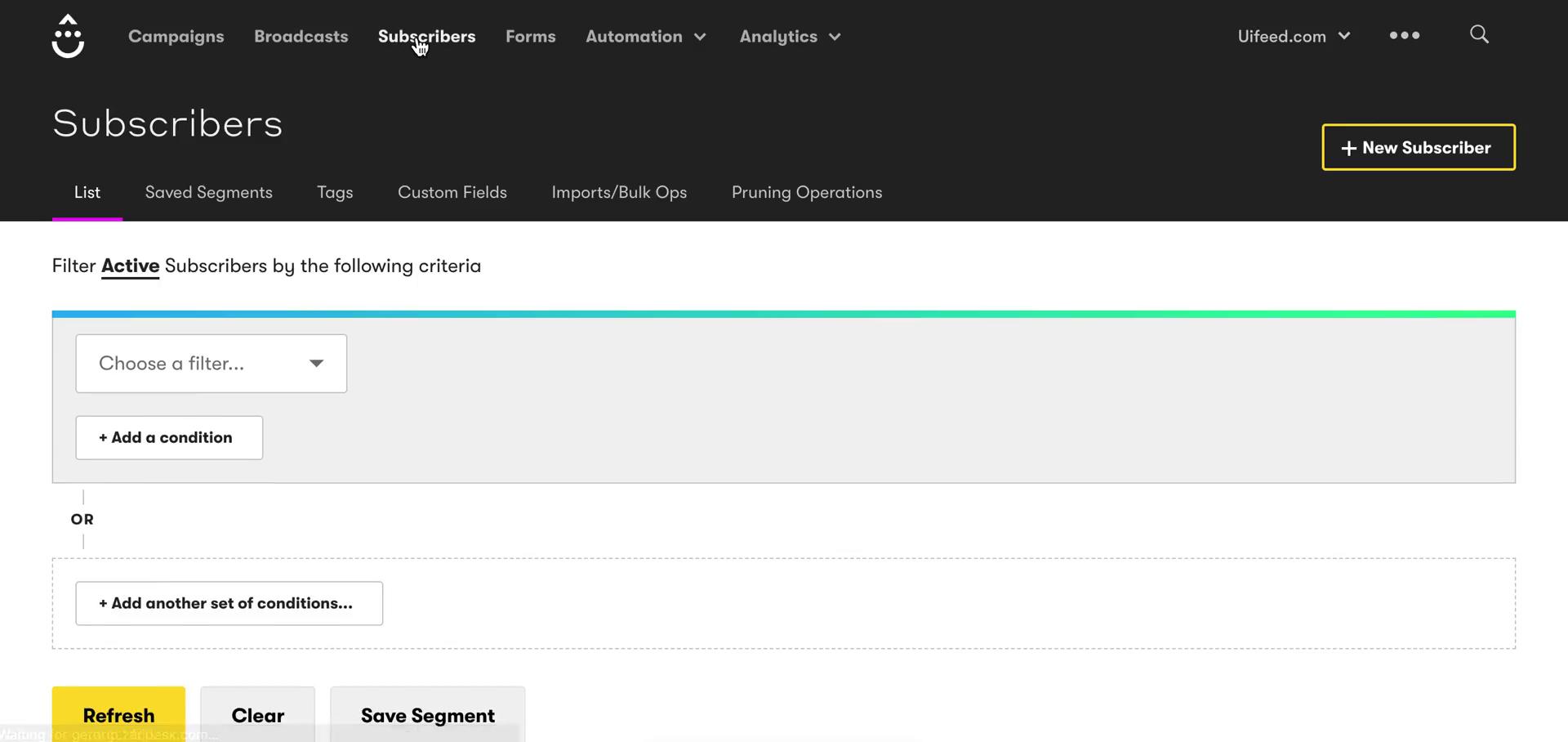At the top of the page, there is an up arrow icon followed by three horizontal dots and a half-circle symbol. Moving to the right, the words "Campaigns" and "Broadcasts" are displayed in gray, while "Subscribers" appears in white, highlighted by a pointing hand. Further right, you’ll find "Forums," "Automation," and "Analytics," all in gray text.

Directly below, there is a navigation bar with a down arrow, three horizontal dots, and a magnifying glass icon, accompanied by the word "Subscribers" in larger letters. To the right of this is an outlined horizontal rectangle labeled "Plus New Subscriber."

Underneath this section, there are six tabs within a black box: "List," "Saved Segments," "Tags," "Custom Fields," "Import/ Bulk Ops," and "Printing Operations." Below these tabs, there is a filter section titled "Active Subscribers by Following Criteria." This is indicated by a line transitioning from teal to green over a gray background. 

Additionally, there is a gray rectangle with a white rectangle below it labeled "Choose Filter."